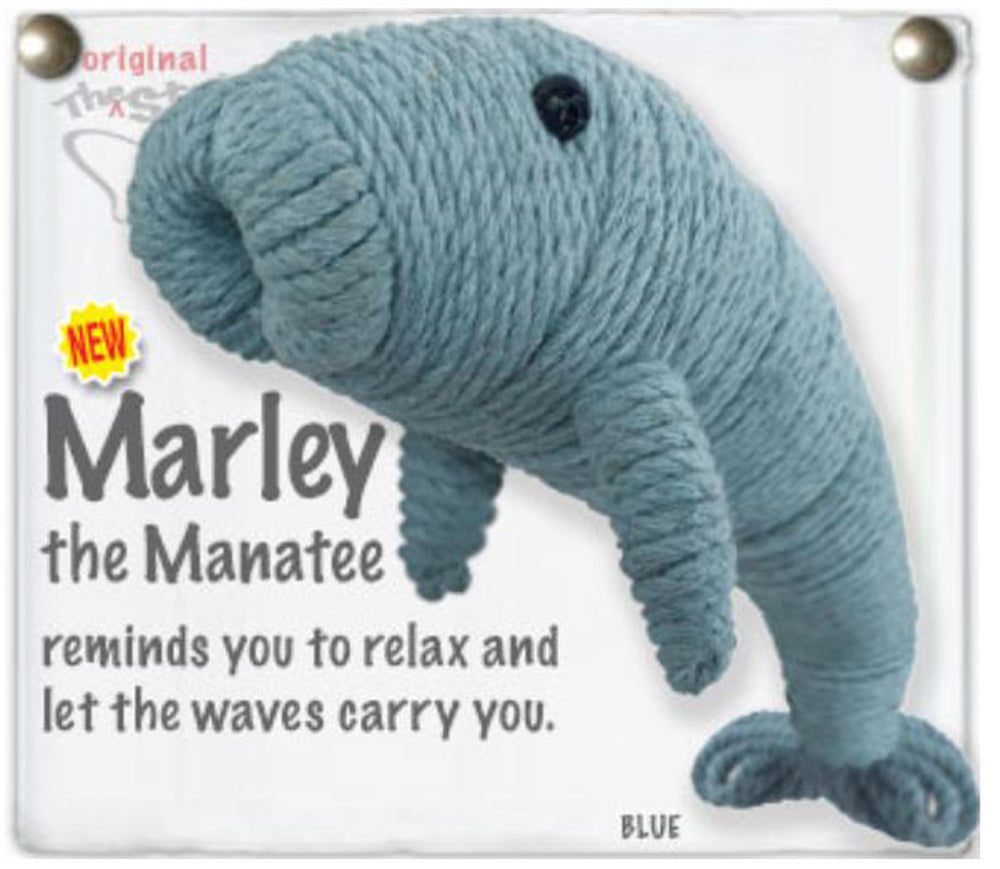This image, photographed indoors, showcases the cover of a toy advertisement featuring "Marley the Manatee," a doll fashioned from blue yarn. The manatee, complete with black eyes, a front mouth, two flippers, and a small tail, is positioned diagonally from the bottom right corner to the top left corner of the image. At the top left corner, partially obscured by the manatee, the text "original" in pink letters followed by "ST" in gray is visible, possibly indicating the name of the store. Below this, a yellow star with red writing announces "NEW." The main text in gray reads, "Marley the manatee reminds you to relax and let the waves carry you," with the word "blue" in the same gray font at the bottom center-right. The image appears to be pinned using brass-colored pins at the top left and right corners, suggesting it's an advertisement card, although the background wall is not visible.